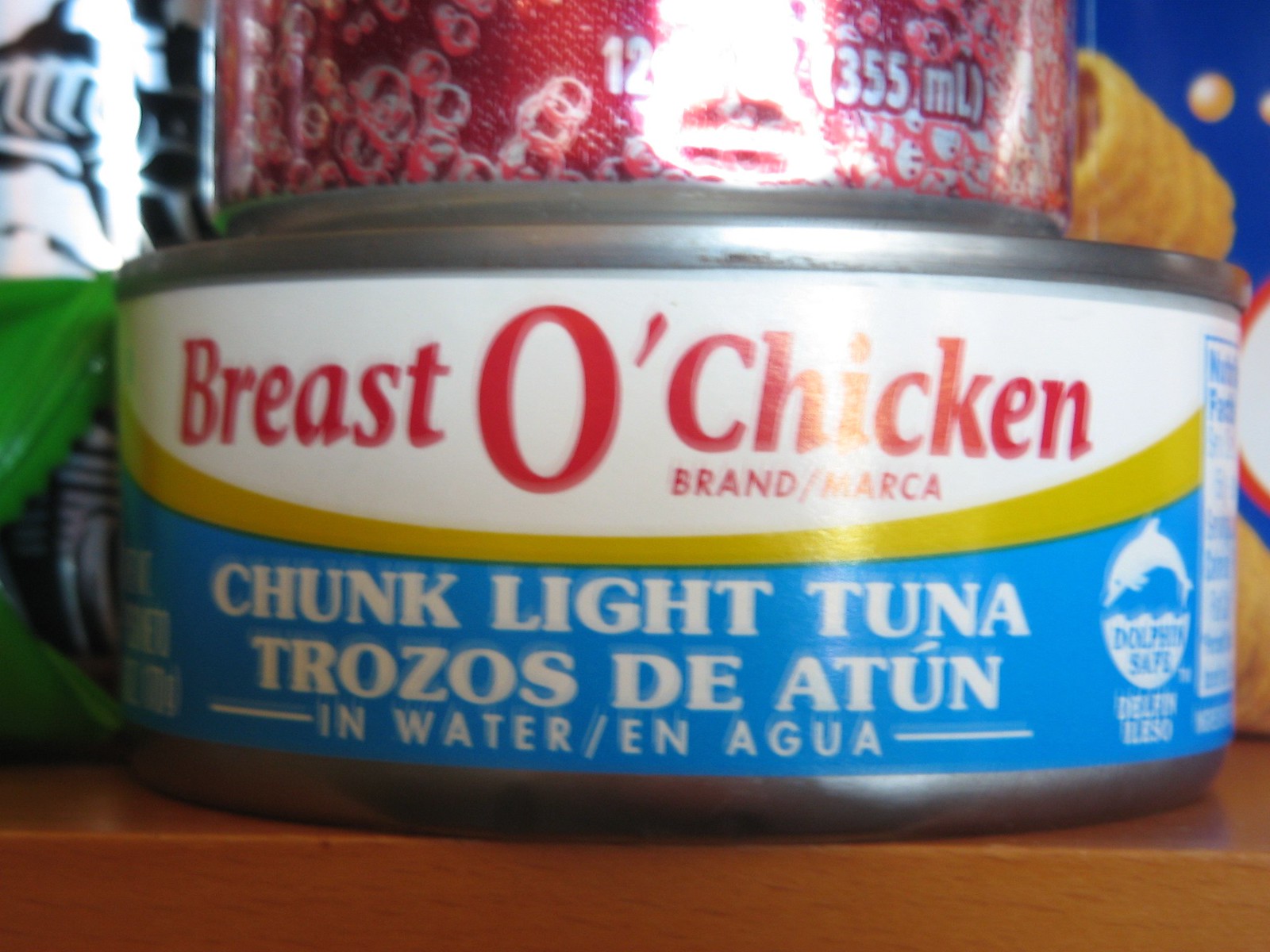The image captures a can of “Breast O' Chicken” Chunk Light Tuna prominently placed on a brown wooden counter. The can features a distinct label with a curved half-circle at the top in white with a yellow edge, bearing the brand name “Breast O' Chicken” in bold red letters. The majority of the label is blue, displaying “Chunk Light Tuna” and “Trozos de Atun” in white text along with “in water” and “en agua.” To the right of the label is a small white circle with a blue dolphin icon and the phrase “Dolphin Safe.” Behind the can, on the left, there is a blurred green and white object and a partially visible red aluminum can with “355 ml” written at the bottom, likely a soda can with white bubbles. On the right-hand side of the frame, there is a dark blue area in the upper right corner with some yellow below it, resembling another package or item, adding to the context of a likely kitchen or pantry setting.